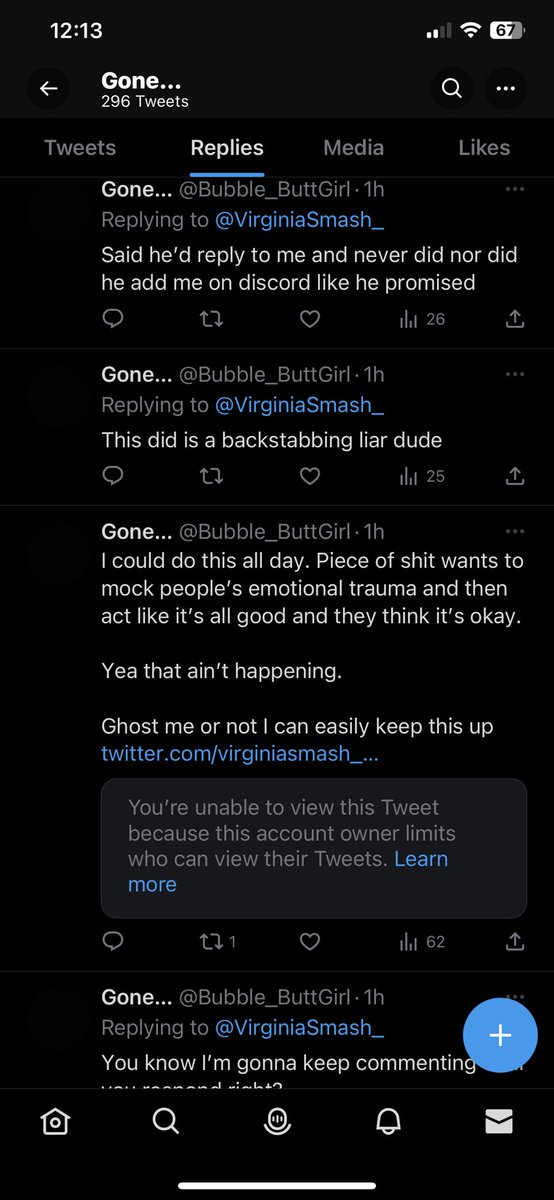A Twitter post displayed on a dark-themed interface with white font. The user, whose name is partially obscured with just "gone…" visible and a username "bubble_butt_girl," is in the "Replies" section of their profile. She is replying to a user named Virginia Smash, expressing frustration that he promised to reply to her and add her on Discord but failed to do so, calling him a "backstabbing liar." She further states to no one in particular her determination to expose those who exploit people's emotional trauma, highlighting her resilience with, "I could do this all day, piece of shit." Additionally, there's a note that some content couldn't be viewed due to restricted access by the tweet's owner. The reply appears to be part of an extended thread of comments, the latest reiterating her intent to keep commenting despite appearing indifferent.